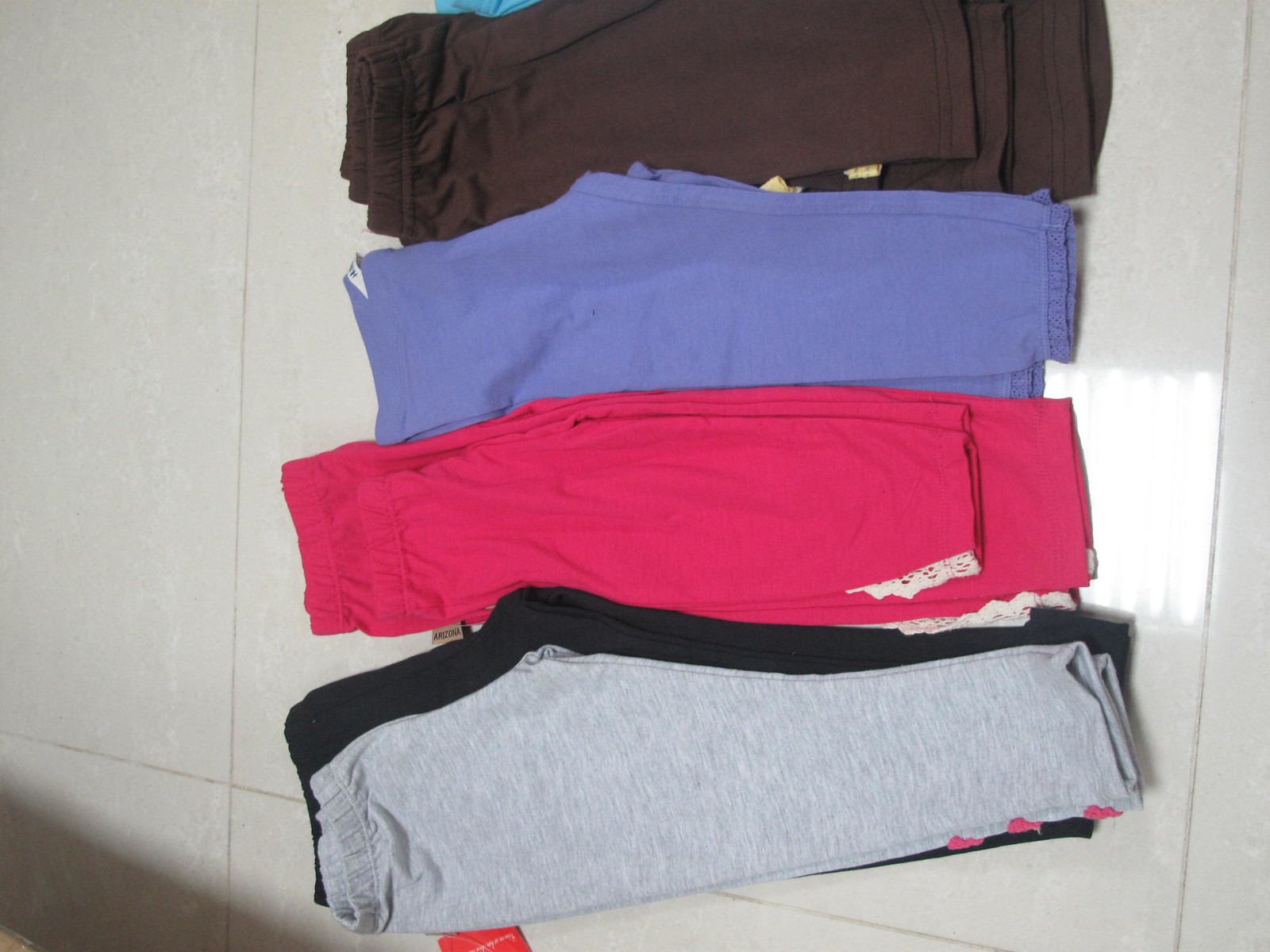In the center of the image, a carefully arranged pile of folded pants sits on a large white tiled floor, with light streaming in from an open window. The pants, likely women's or girls' sweatpants, are organized in neat rows, with each row featuring similar-colored pairs stacked together. The colors vary, including shades of gray, black, pink, light periwinkle blue, dark bluish-purple, and brown, with some colors barely visible beneath the others. Notably, bits of intricate lace trim embellish some pants, suggesting they are designed for girls. Among the stacks, a reddish-pink pair prominently displays an "Arizona" tag on the waistband.